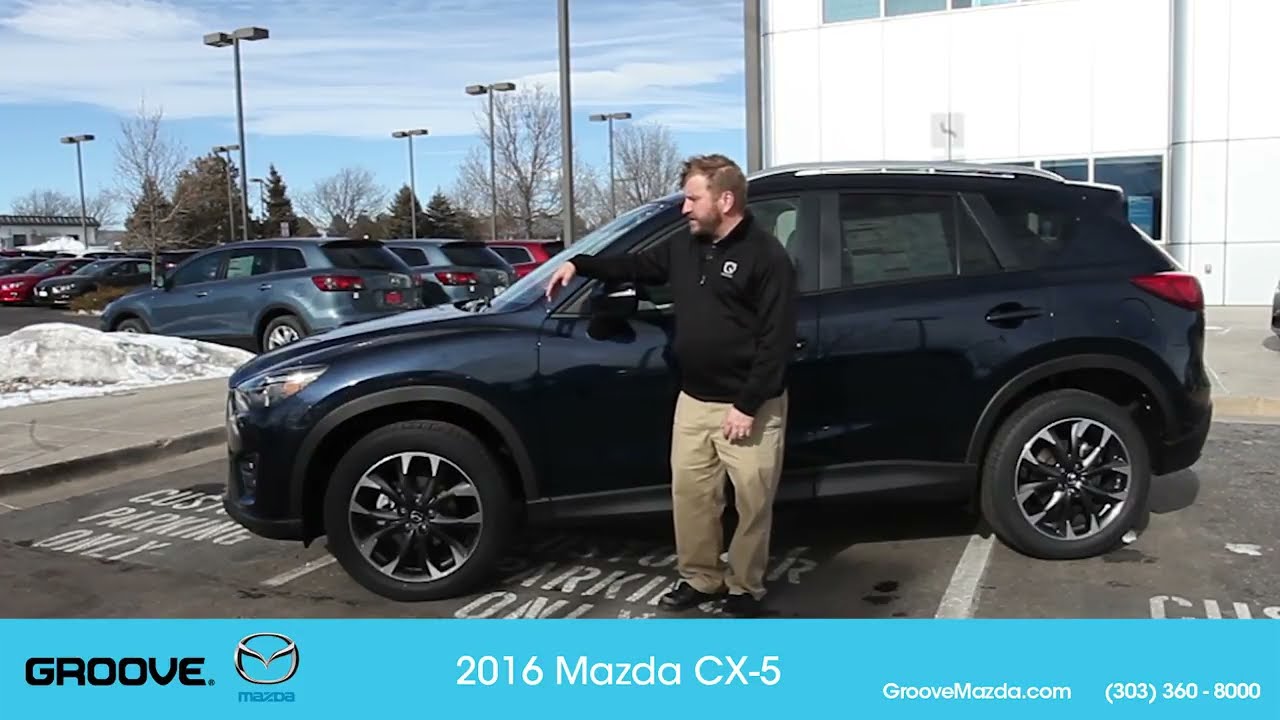This vividly detailed advertisement showcases a sleek 2016 black Mazda CX-5 prominently positioned in the center of a dealership parking lot. The scene is set in winter, with snow visible on the ground to the left and leafless trees in the background. A man stands beside the driver's side door, his right arm resting on the mirror. He is light-skinned and sports short hair, a beard, and a mustache. Dressed in a black jacket with a white patch on the upper chest, long khaki pants, and dark shoes, the man appears to be a representative from the dealership.

In the background, other cars are visible, emphasizing the dealership environment. The pavement in the foreground clearly reads "Customer Parking Only" in white letters. A blue border at the bottom of the poster features the Groove Mazda logo on the left, with “Groove” in black text and “Mazda” in blue alongside the brand's symbol. The right side of the border lists the dealership's website, GrooveMazda.com, and their phone number, 303-360-8000, in white text, underscoring the dealership's branding and contact information.